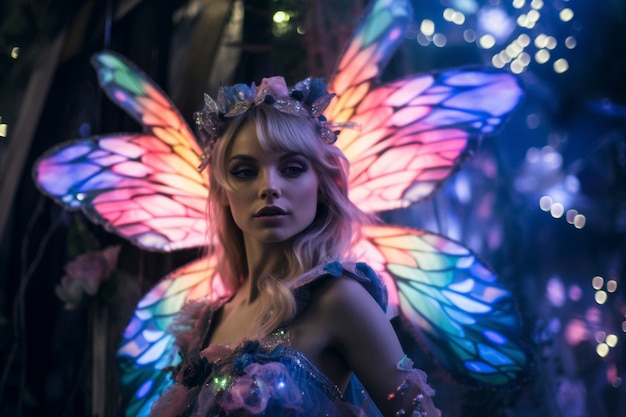The image depicts a blonde woman with long, flowing hair, adorned with a crown crafted from flowers. She is dressed in a wispy, rainbow-colored sleeveless dress and wears large, vibrant butterfly wings in shades of pink, orange, green, purple, and blue. Her arms are decorated with bangles. The woman stands against a dense forest backdrop, with sunlight filtering through the trees, creating a dreamy atmosphere filled with glittering lights in various colors, including white, purple, and yellow. Her expression is sullen as she gazes towards the bottom left, possibly at something or someone off-camera, evoking a sense of mystery. The photograph’s left side is dark and blurry, adding to the ethereal and enchanting quality of the scene, which suggests she might be cosplaying as a fairy.